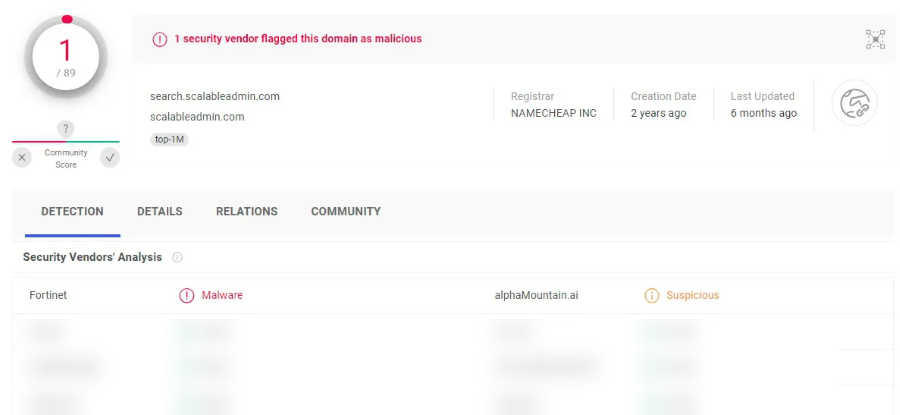This image appears to depict a security report screen, possibly from a service similar to McAfee's. The background predominantly features shades of gray and white. 

- At the top left, there's a white circle containing a red "1" with a gray forward slash followed by "89". 
- Below this circle, the text "Community Score" is displayed, accompanied by a grayed-out question mark at the top.
- A red line is seen extending to the left, and a green line extends to the right of the "Community Score" text.
- Just underneath these lines are two gray circles: one with an "X" and the other with a checkmark, with "Community Score" situated between them.

Above these elements, within a grayed-out rectangle, there's an alert message in red font stating, "1 Security vendor flagged this domain as malicious."

Further down, there's text displaying a URL: "SCALABLEADMIN.com" along with its repetition, formatted as "SCALABLE-Admin.com". Additional information is provided, including "top 10 - 1M", and details about the registrar, creation date, and the domain's last update.